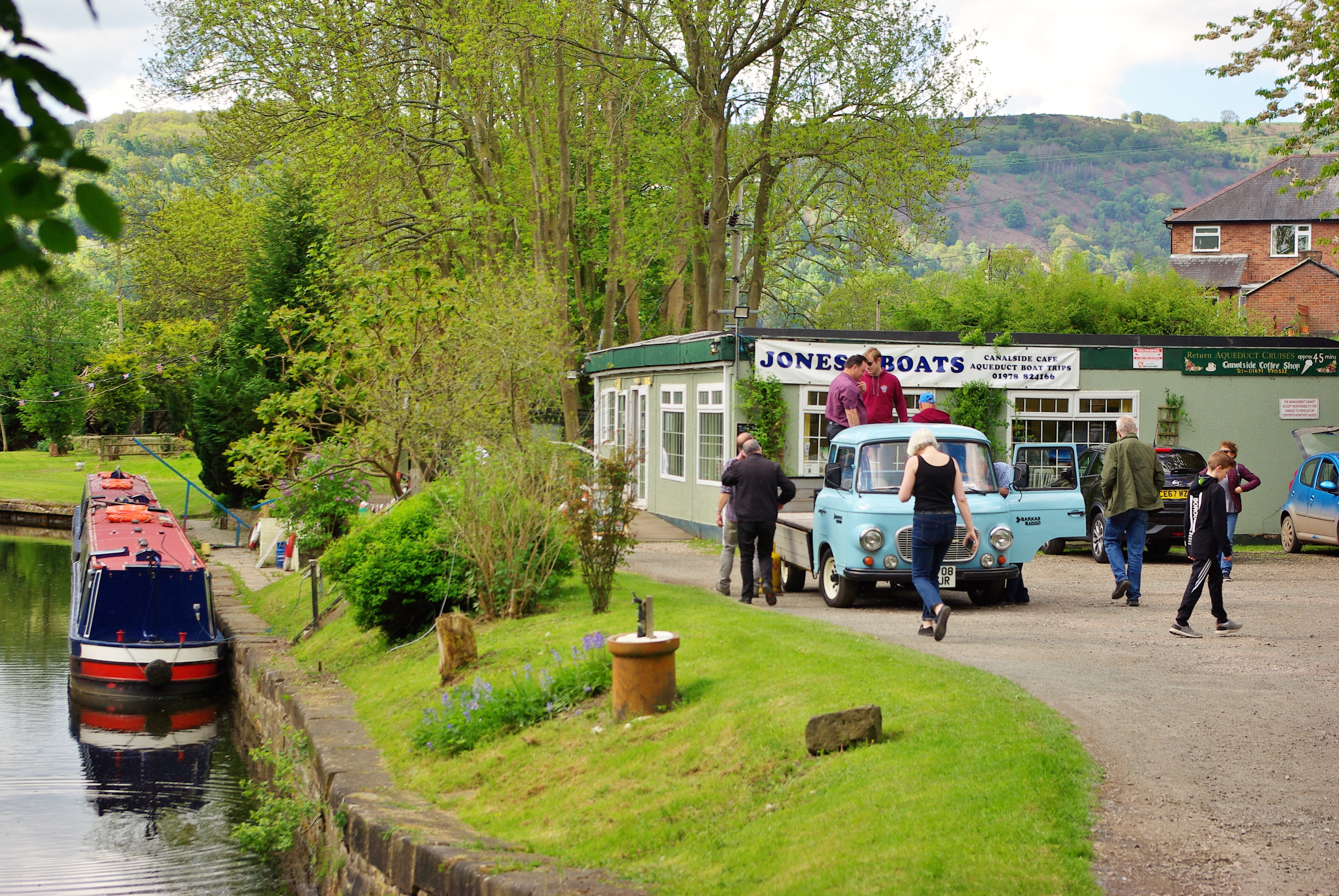The photograph captures a picturesque scene at a lakeside tour and fishing area. The backdrop features a cloth banner with "Jones Boats" emblazoned on it, suspended over a quaint, one-story building where groups of people are gathered. The setting is lush and verdant, surrounded by vibrant green foliage, mountains, and clear waters, indicative of a scenic resort area. A distinctive blue truck, with an open bed, is parked nearby, adding a rustic charm to the scene. The license plates on the vehicles hint at a foreign locale, possibly a charming small town in Wales, Scotland, or Ireland. The image beautifully encapsulates the serene and inviting atmosphere of the locale, making it difficult to distinguish whether it’s an advertisement or a candid snapshot.